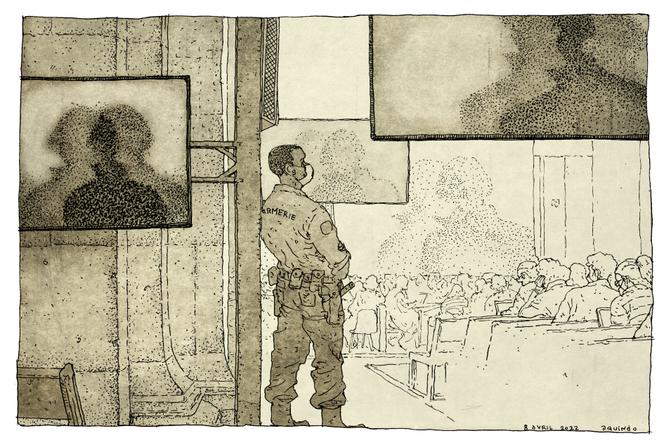The image is a highly detailed black and white sketch, possibly drawn in pencil with some elements that could be watercolor or ink. On the left side, there's a wall featuring a rectangular picture with abstract, silhouette-like designs. To the right of this image is a man wearing a police or security uniform, identifiable by the guns and various equipment on his belt. He is leaning against an iron structure extending from the top of the image. The man, whose face is masked, appears to be watching over a group of people seated on benches in a galley area, which suggests the setting might be a courtroom, church, or classroom. Behind the seated individuals, three screen-like objects display silhouettes and shadowy figures. The overall color tones of the sketch are brownish and gray, and the piece is signed by the artist in the bottom right corner, though the signature is too small to read clearly.